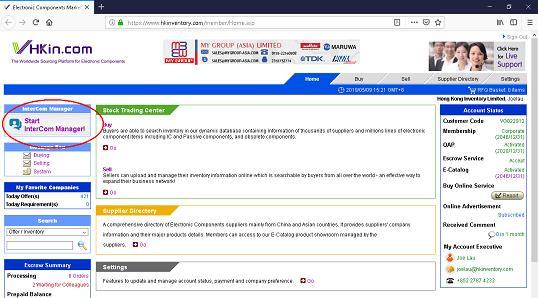This is a detailed caption for the provided image:

"The webpage from vhkn.com features a top navigation bar with a left-facing arrow, a refresh button, a home button, and a search bar, followed by a hamburger menu on the far right along with two indistinct icons. Below the navigation bar, there is a promotional ad for a group called 'My Group - Limited'. This is followed by five tabs, with only the last tab, labeled 'Setup,' being readable. The left column highlights options with a red circle around 'Start,' 'Intercom Management,' and 'Intercom,' along with check boxes beneath that, though the exact details of 'My Competitors' are unclear. The middle column begins with a banner that likely reads 'Stack Trading Center,' followed by a yellow 'Support Directory' banner, and a grey 'Settings' banner. The right column, seemingly dedicated to 'Account Status,' contains several sections, the last of which is labeled 'My Account Executive,' though the other details are not legible."